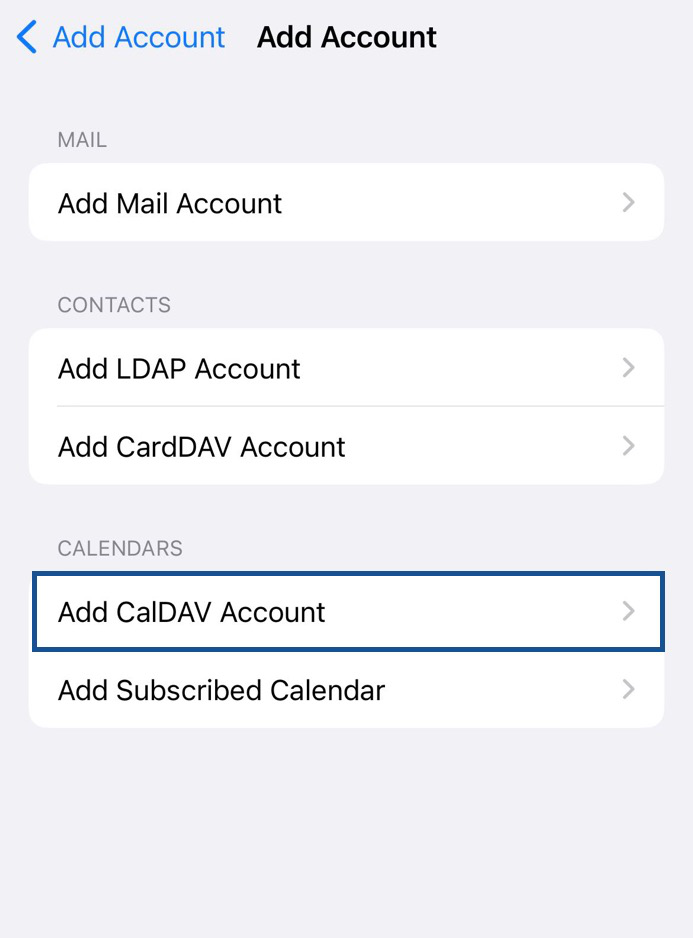This is an "Add Account" page for a mail application, featuring a gray background. At the top left, there is a left-pointing arrow followed by the text "Add Account" in blue. Below that, the heading "Add Account" is displayed in black font.

The page is divided into sections as follows:

1. **Mail Section**:
   - "Mail" text is followed by a white selection box labeled "Add Mail Account," accompanied by a gray right-pointing arrow.

2. **Contacts Section**:
   - Options include "Add LDAP Account" and "Add CardDAV Account," both with gray arrows pointing to the right.

3. **Calendars Section**:
   - Contains "Add CalDAV Account," which is highlighted in dark blue, and "Add Subscribed Calendar," each with gray arrows pointing to the right.

These features suggest that the page is designed for adding various types of accounts, including mail, contacts, and calendars, to integrate different functionalities into a single application.